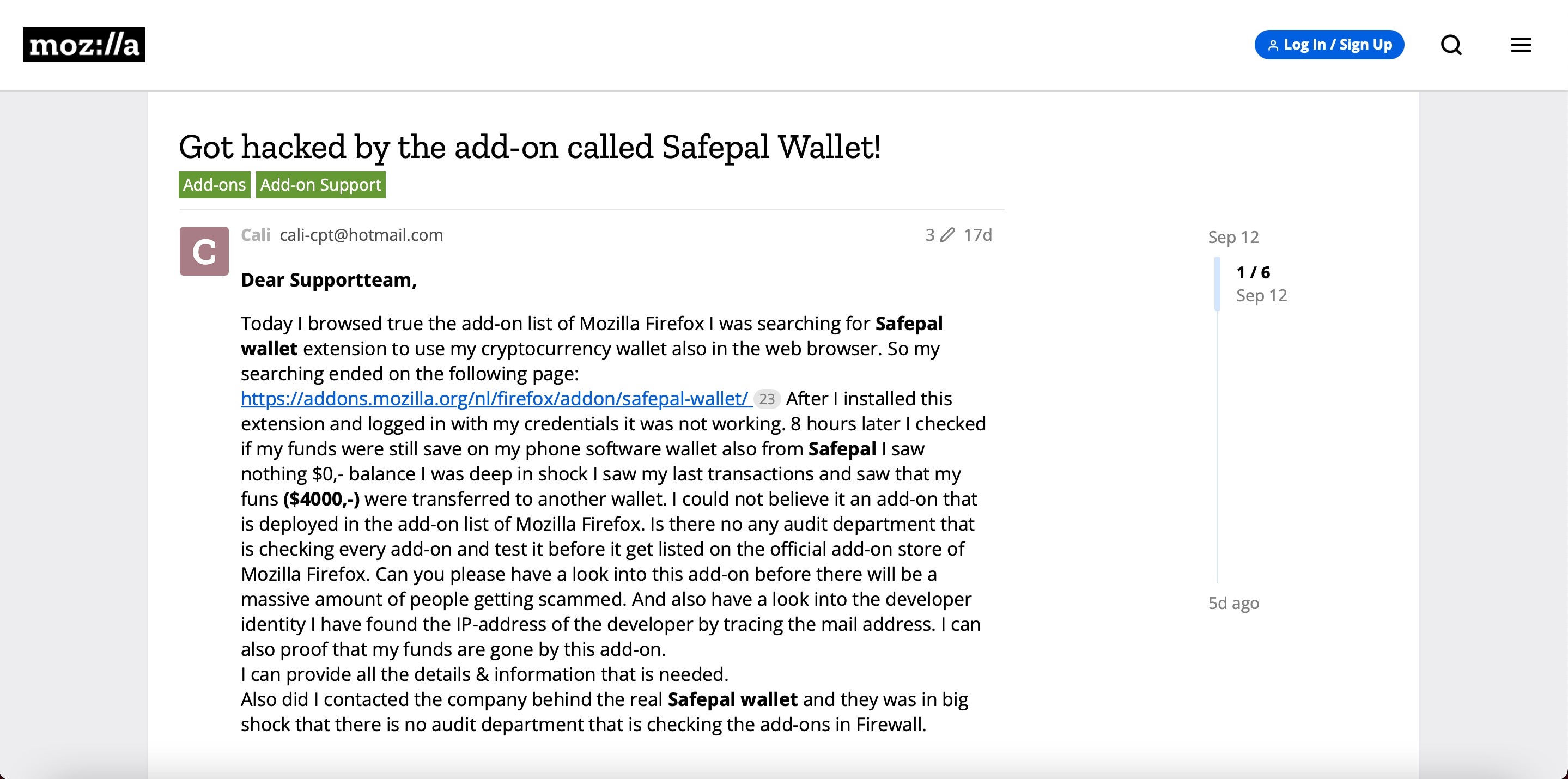**Caption:**

In the upper left corner, a black rectangle with white text reads "Moz://a." The rest of the background is white or gray, with a vertical strip on the left side displaying some text. It states "Got hacked by the add-on called S-SafePal Wallet!" in a bold, alarming manner. Below, there are two green rectangles; one labeled "Add-ons" in white and the other saying "Add-on Support." 

A rose-colored box features the letter "C" in white and an email address, "Kali-CPT@hotmail.com." Following this is a naive yet worried message to the support team:

"Dear support team, today I browsed through the add-on list of Mozilla Firefox. I was searching for the SafePal Wallet extension to use for managing my cryptocurrency wallet in the web browser. My search led me to a specific page (link provided in blue). After installing the extension and logging in with my credentials, I found it non-functional. 
Eight hours later, I checked my SafePal wallet on my phone, only to discover a zero balance. Shockingly, a transaction indicated that my $4,000 had been transferred to another wallet. This incident involves an add-on listed in Mozilla Firefox's add-on repository."